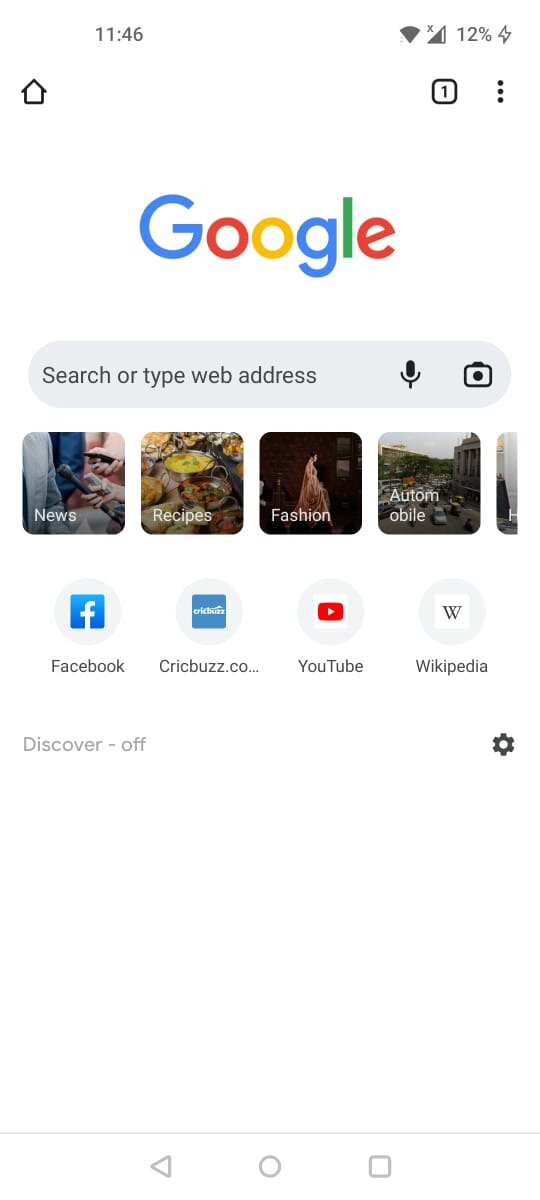This image shows a detailed screenshot of a mobile device interface, likely a smartphone or tablet. The top of the screen displays the time, 11:46, in the upper left corner, alongside the battery indicator at 12% with a charging symbol, and a Wi-Fi connectivity icon.

Dominating the main content area is a white background featuring various elements associated with a Google search page. At the top, the recognizable word "Google" is prominently displayed, below which lies a search box containing the prompt "Search or type web address," accompanied by microphone and camera icons for voice and image search functionality.

Beneath the search box, several category icons with corresponding text labels are visible, including "News," "Recipes," "Fashion," and "Automobile." Further down are four additional icons with their respective labels: "Facebook," "Crickbuzz.com," "YouTube," and "Wikipedia." A gear icon suggesting user settings options is also present.

A section labeled "Discover," which appears to be turned off, lies below this array of icons and categories. The bottom of the screen features the standard navigation icons commonly found on Android devices: a left-pointing arrow for the back button, a central home button, and a square button for accessing the multi-window view or recent apps.

In summary, this screenshot captures the Google search page interface on a mobile device, complete with various functional and navigational elements indicative of a typical user's digital environment.